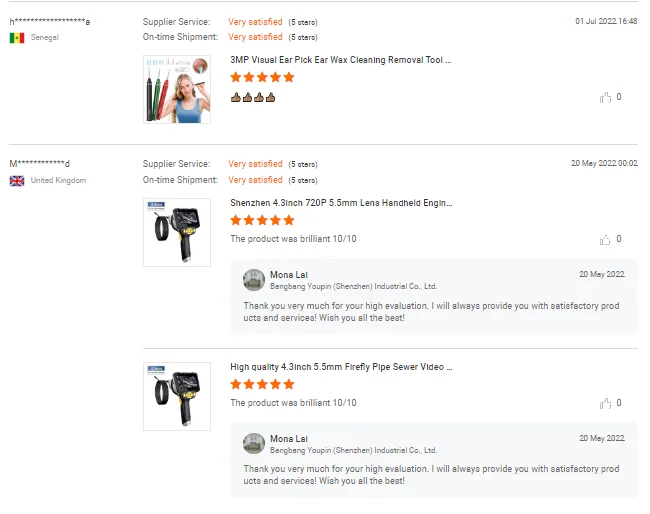This image appears to be a screenshot from a product review section on an e-commerce website. At first glance, the names of the reviewers have been censored for privacy, but their countries are visible along with the corresponding flags. 

The first review is from a customer in Senegal, marked with Senegal’s flag. The customer rated the supplier service as "very satisfied" with five stars and similarly rated the on-time shipment with five stars. The product reviewed is a "3 MP Visual Ear Pick Earwax Cleaning Removal Tool," which is depicted in an accompanying image. The customer left a very positive review, indicated by four thumbs up, and the review was posted on July 1, 2022, at 16:48 PM.

The second review is from a customer in the United Kingdom, indicated by the UK flag. The reviewer rated the supplier service and on-time shipment both with five stars. The reviewed product is a "Shenzhen 4.3 Inch 720P 5.5 mm Lina Handheld Engine," also shown in an image. The review describes the product as brilliant and gives it a perfect score of 10 out of 10. Additionally, the reviewer thanked "Mona Lao bang bang you pin Shenzhen Industrial Co Ltd." for their high evaluation and expressed a commitment to providing satisfactory products and services, ending with best wishes to the customer.